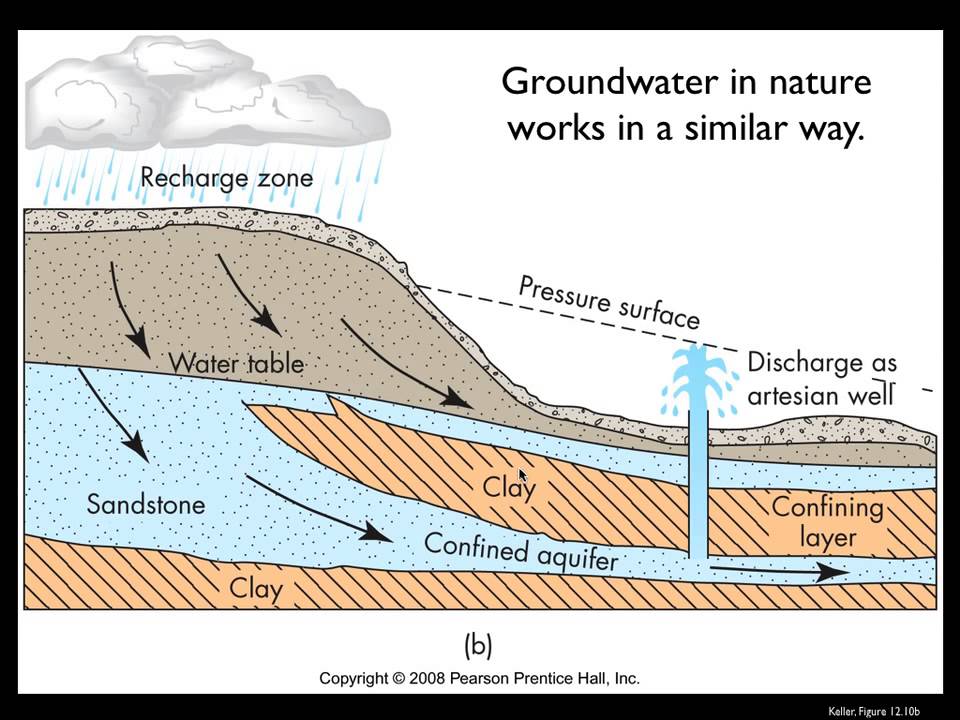This detailed diagram, likely from an Earth Sciences textbook, is titled "Groundwater in Nature Works in a Similar Way" and was created by Pearson Prentice Hall Incorporated (copyright 2008). The illustration shows the process of groundwater movement, beginning with a rain cloud positioned in the upper left corner, labeled as the recharge zone, from which rain descends onto the ground. The background is predominantly white, with various colors used to differentiate geological layers and processes.

The ground is depicted in cross-section, showing several distinct layers. At the surface, earth layers are illustrated in shades of brown. Arrows indicate the downward movement of water through the soil into the water table, a brown layer that marks the top of the groundwater zone. Below the water table lies a blue-tinted layer of sandstone. The diagram shows water permeating through this sandstone into a confined aquifer, a narrow, tubular area trapped between two clay layers. These clay layers, rendered in a taupe-gray hue, serve as barriers that compress and trap water within the sandstone.

Additionally, the diagram features an artesian well, where water from the confined aquifer is discharged. This well is shown with water shooting up through the clay and sandstone layers, the water table, and finally emerging at the earth's surface. The image also includes a dotted line labeled "pressure surface," indicating the pressure conditions driving water flow within the aquifer system. Overall, the diagram effectively illustrates the natural process of groundwater recharge, storage, and discharge, with clear visual representations and labels to enhance understanding.